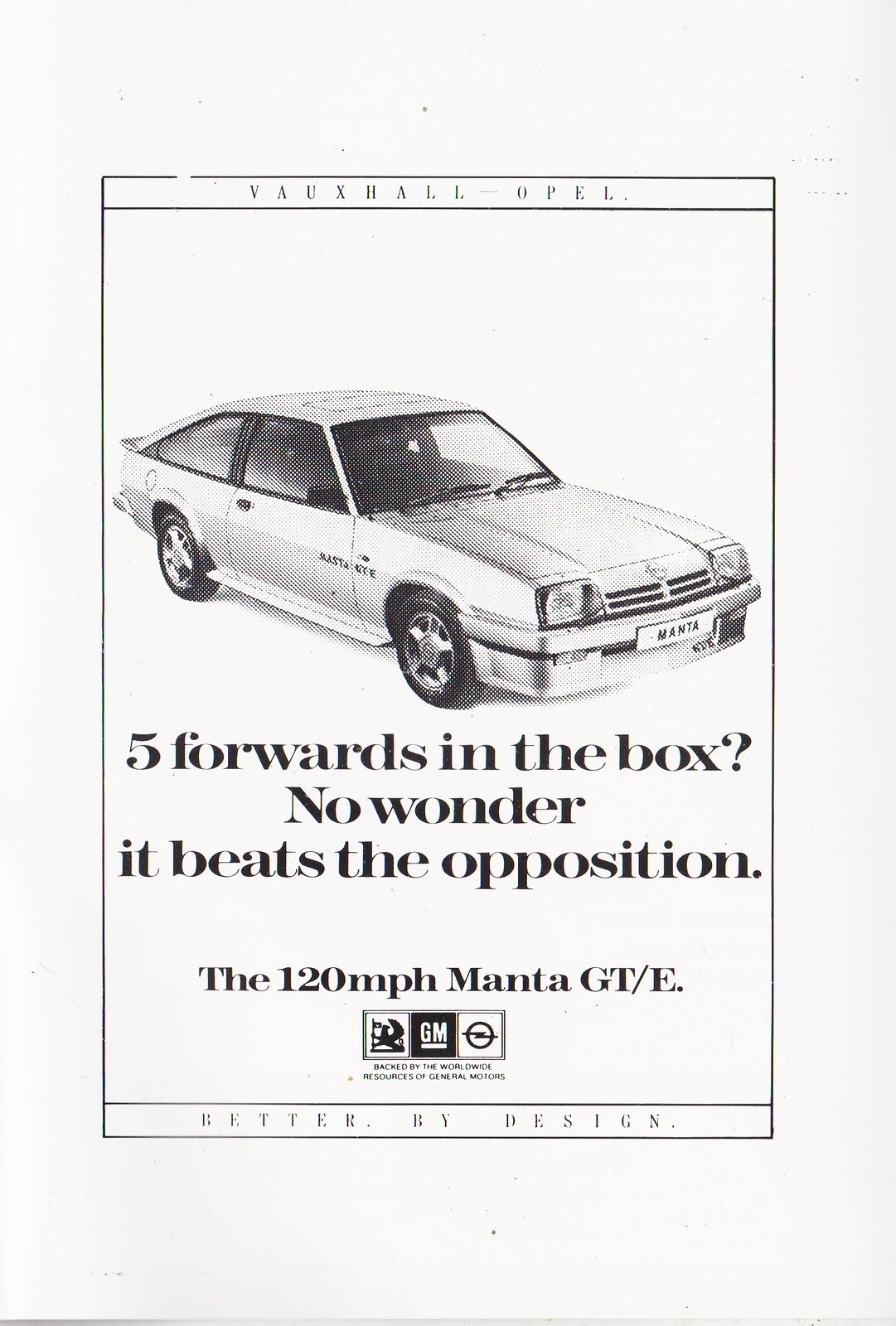The image is a black-and-white vintage advertisement, possibly from a magazine or booklet cover, promoting the Vauxhall Opel Manta GT/E. At the very top, "Vauxhall Opel" is displayed in small black text. The main feature is a sleek, two-door coupe positioned with its front towards the right side, showcasing its passenger side to the camera. The car appears to be from the 1980s, with two headlights and bearing the license plate "Manta." The text "Five forwards in the box. No wonder it beats the opposition." is prominently displayed below the vehicle, followed by "The 120 MPH Manta GT/E" in large black text. Further down, there's a black square logo with 'GM' for General Motors and two additional logos: one with a griffin holding a flag and another with a lightning bolt within a circle. Below these, the slogan "Backed by the worldwide resources of General Motors" can be made out in fine print, leading to the final tagline, "Better by Design." The entire ad is framed by a black rectangular border against a plain white background.